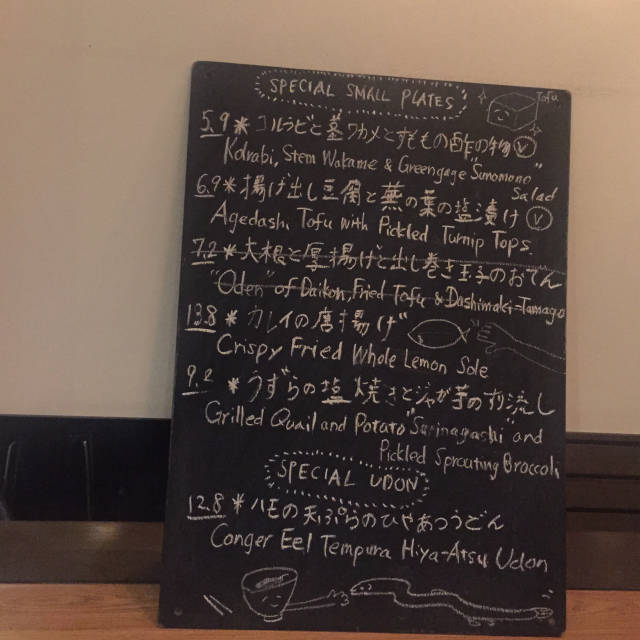This is an image of a slender, vertically-oriented chalkboard commonly used in restaurants to display daily specials. The chalkboard, featuring meticulously written items in white chalk, is titled at the top with "Special Small Plates" and "Special Undone" towards the bottom. It leans at a slight angle, resting its bottom edge on a table and its top part against a white wall with a lower section painted black. The angled positioning of the chalkboard adds a casual and inviting touch to the dining atmosphere, making the day's specials easily readable for patrons.